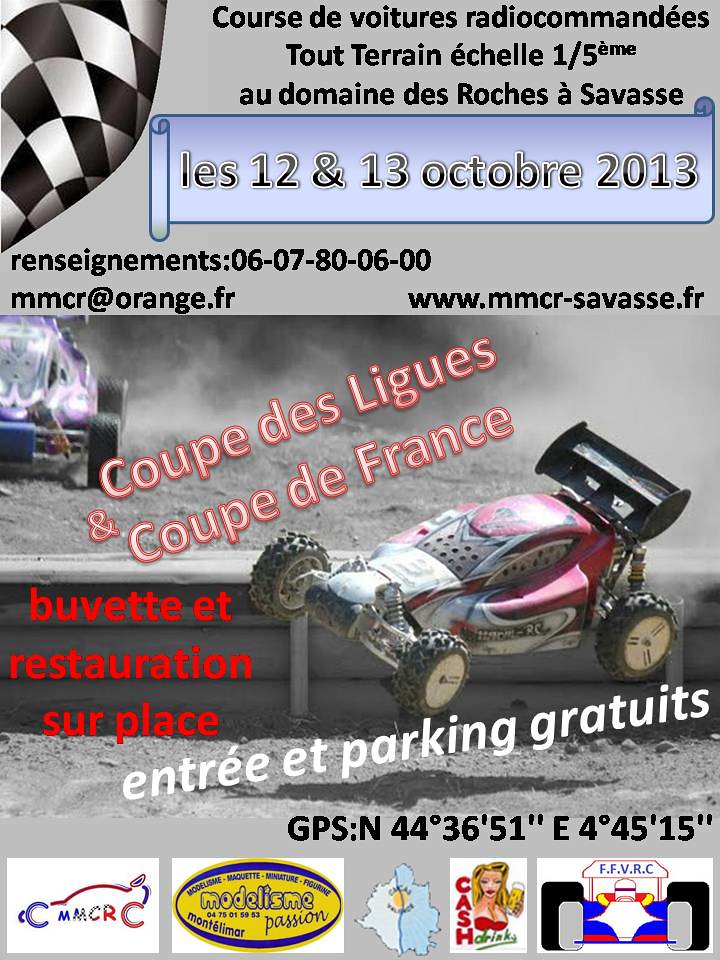Join us for an exhilarating off-road RC car racing event in Savas, Roche on October 12th and 13th, 2013! The flyer, in French, announces the 'Cours de Voiture' with details of the 'Coupe de Ligue' and 'Coupe de France'. An action-packed image in the center showcases a red RC car soaring mid-air between two track levels, while a purple and silver RC car trails closely behind. Sponsors and event organizers are listed at the bottom of the flyer, including GPS coordinates (North 44° 36' 51", East 4° 45' 15"). For more information, contact the organizers via email at mmcr@orange.fr or visit the website www.mmcr-savassse.fr.